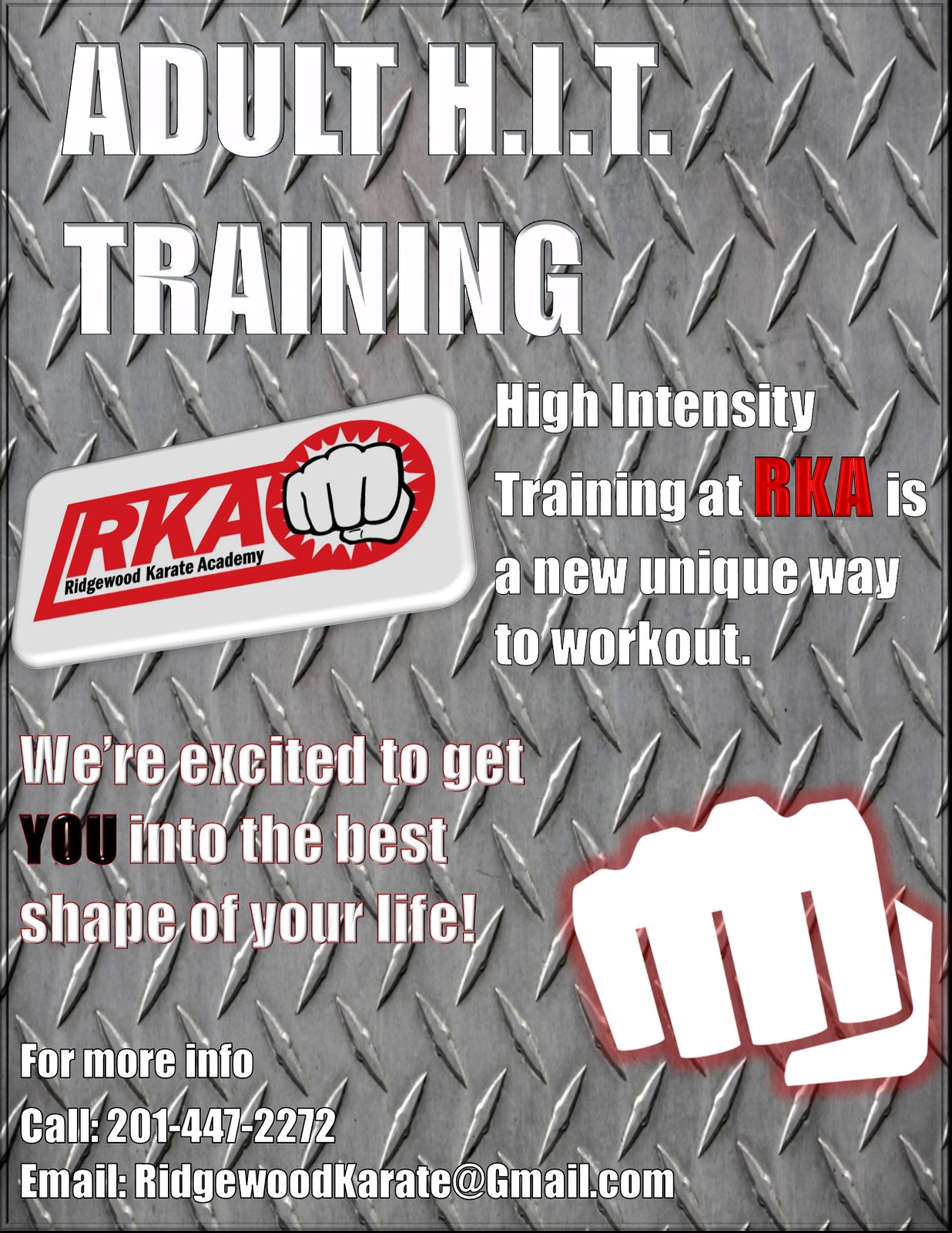The image presents a promotional flyer for "Adult H.I.T. Training" (High Intensity Training) at Ridgewood Karate Academy (RKA). The background is textured with diamond plate metal, commonly found in pickup trucks. At the top, in bold white capital letters, are the words "A.D.U.L.T H.I.T. T.R.A.I.N.I.N.G," followed by a logo featuring a white rectangle with rounded corners. Inside the rectangle, a red rectangle contains the acronym "RKA" in large letters, with "Ridgewood Karate Academy" written below in smaller text. To the right of this is a red circle with a fist punching effect. Additionally, the flyer states in bold red text, "High Intensity Training at RKA is a new, unique way to work out." Below this, it says in black, "We're excited to get YOU into the best shape of your life," with "YOU" emphasized. The bottom left corner displays contact information: "For more info, call 201-447-2272 or email RidgewoodKarate@gmail.com." An image of a stylized fist with a red glow effect decorates the lower right corner.